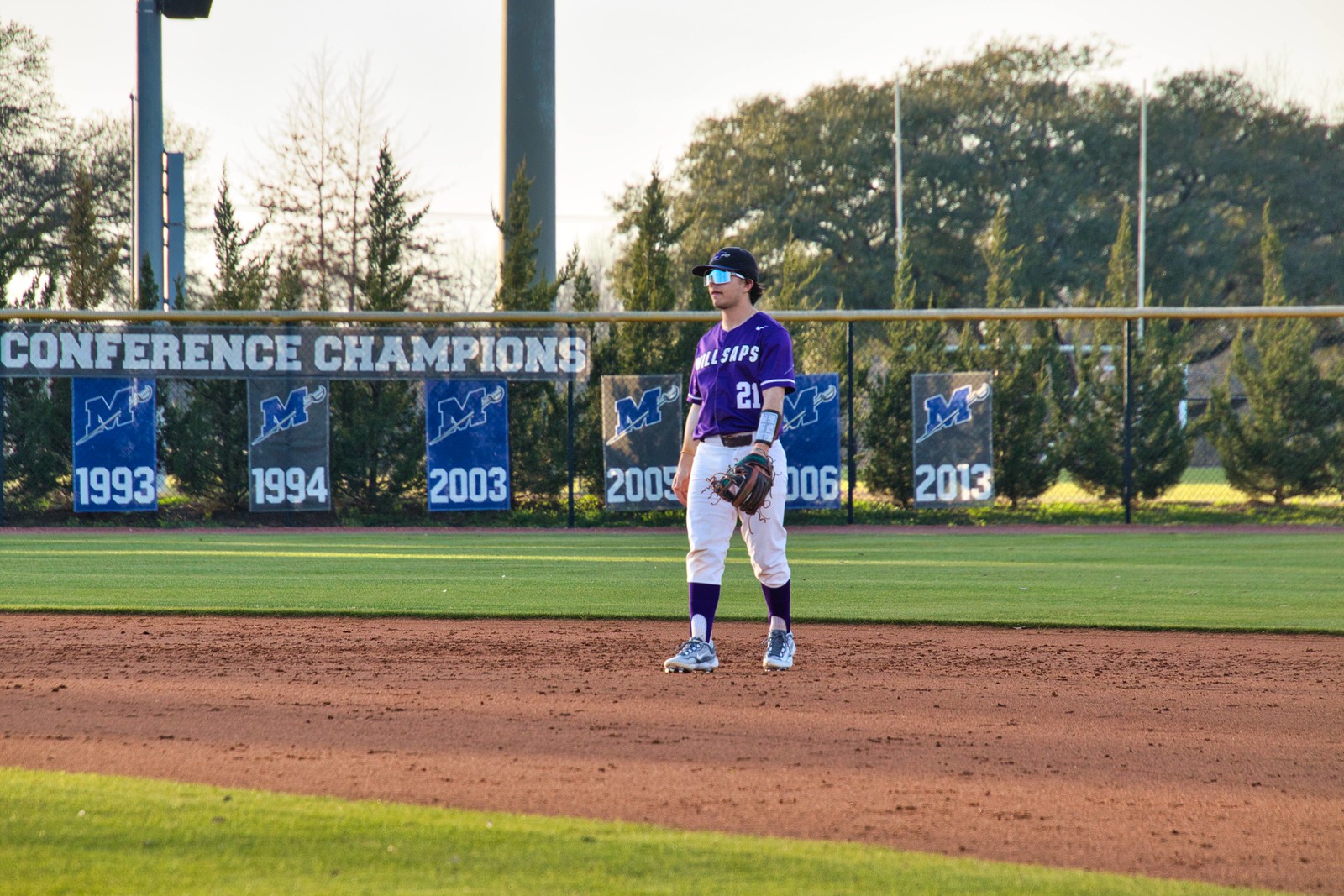In this detailed image, a baseball player is positioned in the outfield, standing on the dirt portion of the field. The backdrop features an array of banners lined up along the outfield fence, celebrating conference champions with an 'M' insignia and the years 1993, 1994, 2003, 2005, 2006, and 2013 displayed on blue or gray backgrounds. To the left of the fence, the words "conference champions" are visible, and behind the fence, a cluster of small trees and tall metal pillars, likely supporting a scoreboard, can be seen, although partially obscured from view.

In the scene, the athlete sports a stylish outfit consisting of a purple jersey adorned with some text and the number 21. He pairs this with white pants and tennis shoes. The player also dons a black baseball cap and mirrored, white-frame sunglasses. A mitt is visible on his right hand. The player's stance indicates motion; his right foot is firmly planted while his left leg trails behind, with the heel slightly lifted. The field itself features a vivid green grass area, bordered by the dirt segments that outline the outfield and baseline.